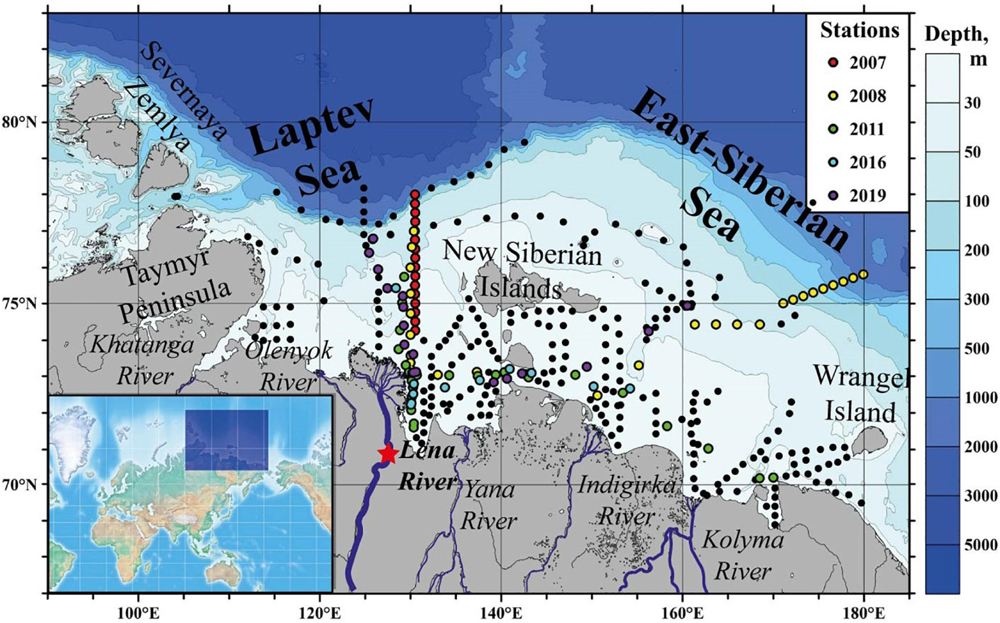This detailed map focuses on the northeastern corner of Canada and the surrounding areas, mainly depicting the Laptev Sea to the left and the East Siberian Sea to the right. The map features various rivers, including the Koloma, Yana, Lena, Kataga, and Olenyok Rivers, with the Lena River marked by a distinctive star. Key landforms such as Wrangel Island, the New Siberian Islands, and the Tamyr Peninsula are also highlighted. A series of colored dots indicate research station locations and the years they were established: red for 2007, yellow for 2008, green for 2011, teal for 2016, and purple for 2019, clustered primarily along the coastlines. The top right corner features a white legend explaining these color codes. Depth variations in the sea are illustrated using an ombre of blue shades. In the bottom left corner, an inset world map within a blue rectangle zooms out to show the focused area. Degrees of latitude and longitude frame the map's borders, providing additional geographical context.